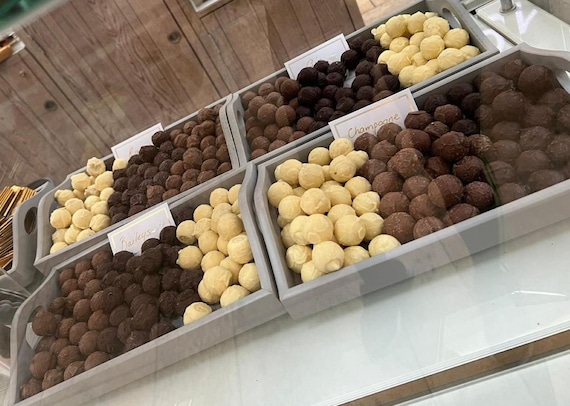The photograph depicts an elegant display of chocolate truffles arranged in four separate, grey trays with handles. Each tray is divided into three sections, showcasing an assortment of white, milk, and dark chocolate truffles. The arrangement is consistent across the trays, with some variation: the back-left tray contains white, dark, and milk truffles; the tray in front of it holds milk, dark, and white truffles; the adjacent tray shows white, milk, and dark truffles; and the back-right tray has a sequence of white, dark, and milk truffles. 

Each tray features a small, white sign with gold lettering on the middle back side. Most of the signs are unreadable except for the front-right tray, where the label clearly reads "champagne." The trays are situated behind a glass case, and the polished, white countertop in front of the display reflects the scene. Additionally, the glass case captures the reflection of someone's legs and feet on the right side of the image. The setup is within a store or market, as suggested by the overall layout and visible brown paneling wall behind the trays.